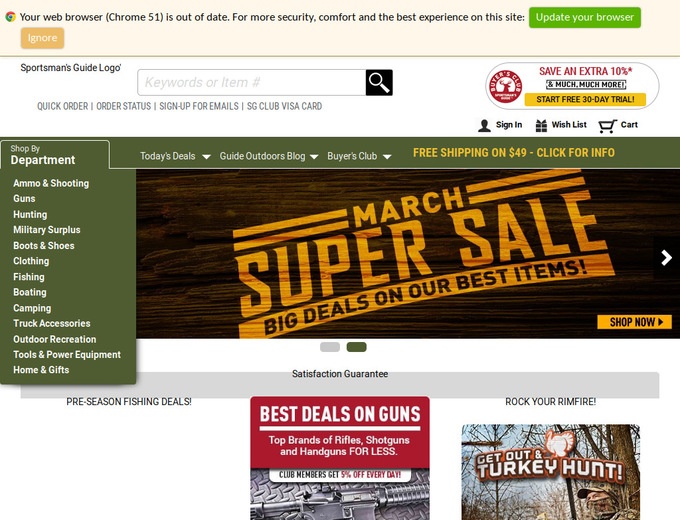A screenshot of the top section of the Sportsman's Guide website, featuring a beige-colored header. At the top, a notification in white text advises that "Your work browser, Chrome 51, is out of date," followed by suggestions to update for better security and experience. This notification is accompanied by green and orange buttons labeled "Update Your Browser" and "Ignore," respectively.

Below the notification, the Sportsman's Guide logo is prominently displayed. Adjacent to the logo is a search bar with a black icon of a magnifying glass. Navigation options include "Quick Order," "Order Status," "Sign Up For Emails," and "SG Club Visa Card." On the right-hand side, a promotional message in green text on a white background encourages visitors to "Save an extra 10% and much more" with a prompt to "Start Free 30-Day Trial." Icons for signing in, wish list, and shopping cart are also present.

Directly underneath, a secondary navigation bar features several headers: "Today's Deals," "Guide Outdoors," "Blog," and "Buyer's Club." Highlighted in bold yellow text on a green background, it announces: "Free Shipping on $49 - Click For Info."

The main promotional banner below showcases the "March Super Sale" with a rustic brown wood background accented by yellow text. In large yellow letters, it proclaims "March Super Sale," while brown text on a yellow background emphasizes "Big Deals on Our Best Items - Shop Now."

On the left side, a sidebar allows users to shop by department, listing categories such as "Ammo & Shooting," "Guns," "Hunting," "Military Supplies," "Boots & Shoes," and more. At the bottom of the sidebar, two clickable images promote "Best Deals on Guns - Top Brands of Rifles, Shotguns, and Handguns for Less" and a "Get Out and Turkey Hunt" campaign.